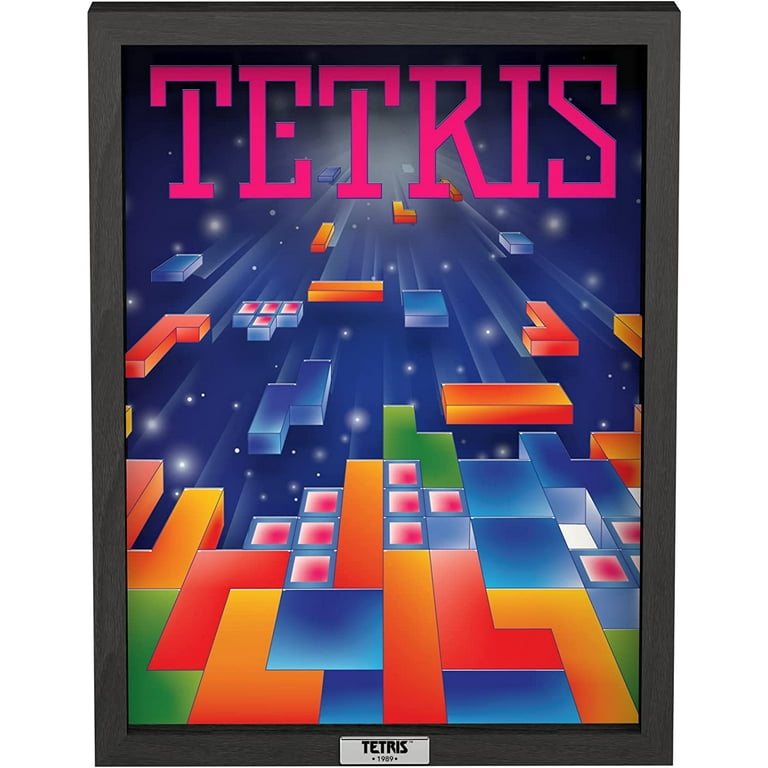The framed poster image is a vertical advertisement for the classic video game Tetris, with a dark brown or light black frame. At the bottom center of the frame, a silver plaque inscribed with "Tetris 1989" provides a nostalgic touch. The poster itself features "Tetris" in bold, magenta pink capital letters at the top. The background is a celestial scene reminiscent of outer space, with a navy blue backdrop adorned with white dots resembling stars. Throughout the image, colorful Tetris pieces—green, yellow, orange, blue, pink, and white—appear to be cascading from the starry sky towards the bottom of the frame, where they are beginning to fill up the game board. The overall effect is a vivid and artistic portrayal of the Tetris game, with pieces transitioning from cosmic elements to their familiar block shapes as they descend, ready to complete the puzzle at the bottom.